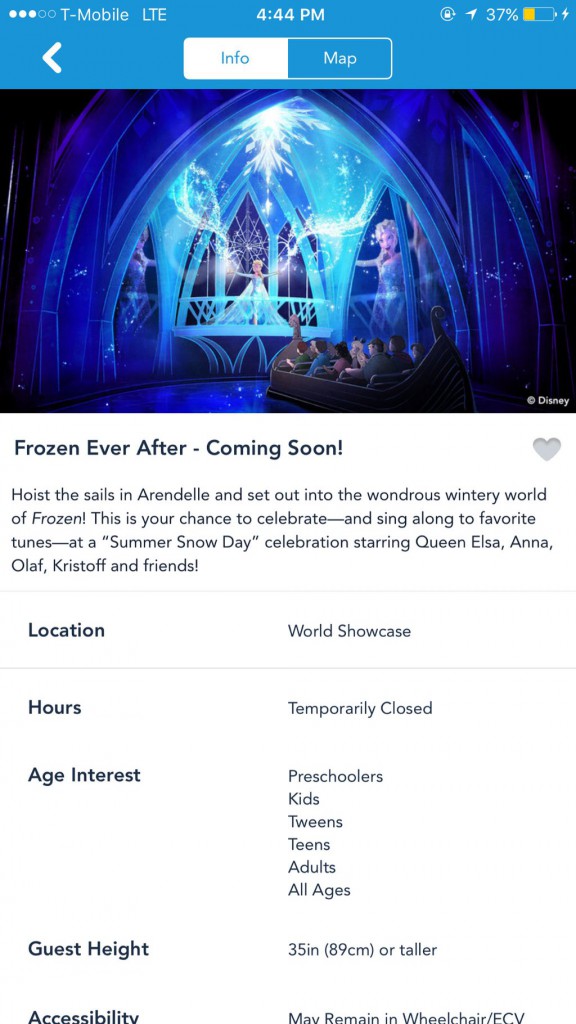A detailed caption for the image could be:

"Searching for an attraction at Disney? Look no further than Frozen Ever After! 'Hoist the sails in,' though I’ve never watched the movie, shouted Arnell, and embarked on a wondrous wintry journey into the world of Frozen. This attraction offers a summer snow day celebration where visitors can sing along to their favorite tunes, starring beloved characters Queen Elsa, Anna, Olaf, Kristoff, and friends. Located in the World Showcase, the attraction’s hours are temporarily closed for now. It's suitable for all ages, from preschoolers to adults, with a minimum guest height requirement of 35 inches (89 cm). At the top of the page, there’s a map showing the location of this enchanting experience. Below the map, a captivating photo showcases the ride as a small boat glides through a wintry landscape, with Elsa majestically perched in the background. The ride features stunning visual effects, whimsical lights, and a cozy atmosphere. The background of the information is blue at the top with the info and map section, transitioning to white with black text. The design is simple but effective, focusing on the vital details and the enchanting photograph of the ride."